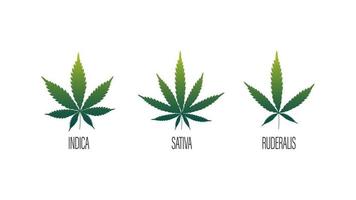The image is a detailed digital artwork showcasing three distinct types of marijuana leaves, each labeled with their respective strain names. On the left, the Indica leaf, with seven broader leaflets, has a gradient color transitioning from darker yellow to light green, ending in dark green. In the middle, the Sativa leaf displays nine thinner leaflets with the same gradient color scheme. On the right, the Ruderalis leaf features five medium-sized leaflets and follows the same color transition. Each leaf is labeled in uppercase, condensed text against a pure white background, emphasizing the visual differences between the strains.